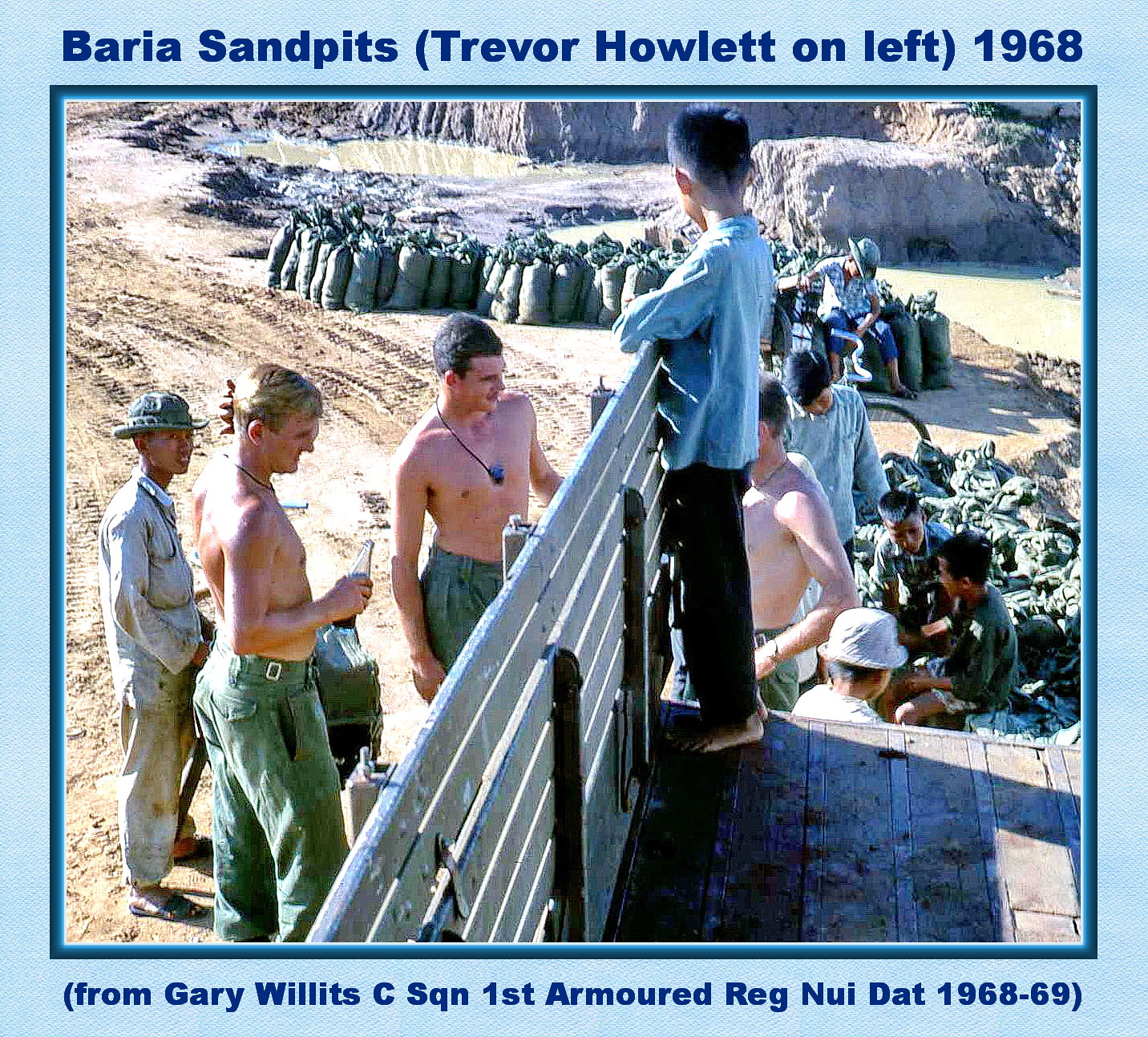In the color photograph from 1968, bordered in powder blue with a navy blue pinstripe, we observe a bustling military scene. Central to the image are two shirtless Caucasian men, each sporting military dog tags and wearing khaki pants. The man in front has blonde hair and holds a bottle, while his dark-haired companion stands nearby. Both individuals focus their attention on a truck, the truck bed partially visible in the lower right of the image.

Beside the truck stands a young Asian boy, barefoot and clad in a blue long-sleeved shirt and black pants, with his face turned away from the camera. Just behind him, another boy, this time Caucasian with short dark hair, can be seen wearing a blue shirt and black pants. Further back in the scene, a man wearing a green boonie hat and light grey clothing sits on the ground. Surrounding them are sandbags, a water or mud pit, and additional young Vietnamese children.

Atop the image, bold blue text reads "Beria Sand Pits (Trevor Howlett on left) 1968." Below, a caption in blueprint states, "(from Gary Willits, CXSQN, first armored, NUIDAT 1968-69)." The detailed setup, expressions, and elements such as the sandbags, duffel bags, and the varied activities give a vivid, historically rich glimpse into this military setting.